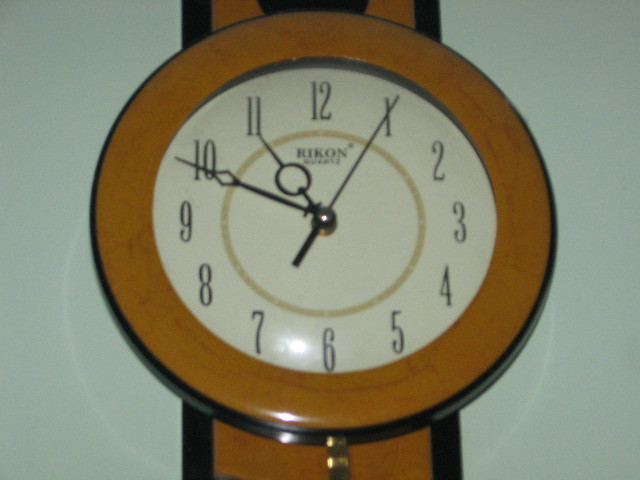A photograph of a clock mounted on a white wall captures an elegantly designed timepiece. The clock features a round face set against a strip of orangey blonde wood, with visible wood grain adding to its rustic charm. The clock face itself is off-white, bordered by a subtle, small gold ring beneath the black numbers and black hands, which all contribute to its classic look. The brand name "RIKON" is prominently displayed on the face. Below the round portion of the clock, there is an additional gold strip that adds a touch of sophistication. A light ring reflects softly on the white wall surrounding the clock, and a slight camera flash is noticeable between the numbers 6 and 7, adding a hint of modernity to the otherwise timeless piece.